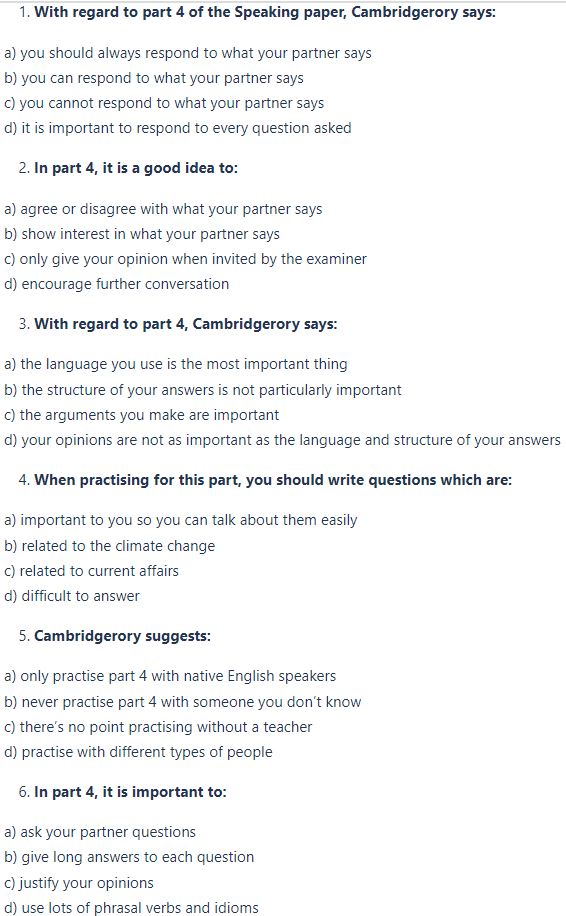**Detailed Caption:**

The screenshot depicts an online questionnaire, likely part of a learning or assessment platform, consisting of six multiple-choice questions (A, B, C, and D) related to Part 4 of the Cambridge Speaking Paper. Each question appears to be designed for practice rather than providing answers immediately. The questions are as follows:

1. "With regard to Part 4 of the speaking paper, Cambridge says:" (options A-D, specific options not visible).
2. "In Part 4, it is a good idea to:" (options A-D, specific options not visible).
3. "With regard to Part 4, Cambridge says:" (options A-D, specific options not visible).
4. "When practicing for this part, you should write questions which are:" (options A-D, specific options not visible).
5. "Cambridge suggests:" (options A-D, specific options not visible).
6. "In Part 4, it is important to:" with detailed options listed as A) ask your partner questions, B) give long answers to each question, C) justify your opinions, and D) use lots of phrasal verbs and idioms.

The screenshot does not indicate the correct answers, suggesting that this questionnaire serves as a worksheet or homework assignment aimed at enhancing understanding and preparation for the specified section of the exam.